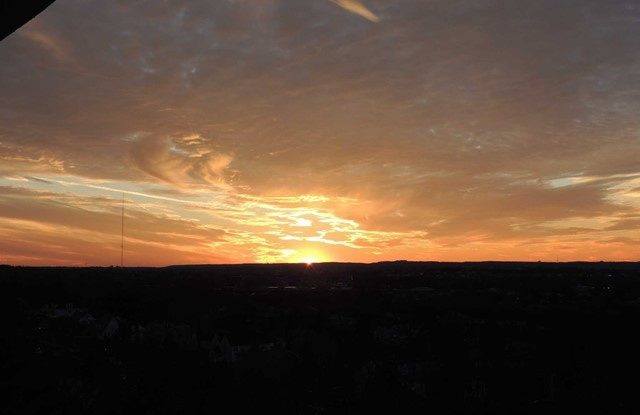This image captures a breathtaking view of a sunset from a high vantage point, possibly from a tall structure, helicopter, or airplane. Dominating the top two-thirds of the composition, an expanse of gray clouds stretches almost across the entire sky, interspersed with glimpses of blue peeking through. As the horizon approaches, the cloud cover decreases, revealing a stunning palette where the blue sky fades into hues of light yellow and white at the horizon. At the very center of this mesmerizing view, the sun, a glowing yellow beacon, emits light through low cloud cover, casting dramatic oranges, yellows, and even some light grayish-pink tones throughout the sky. Below this vivid skyline, the landscape forms a stark contrast, rendered in near-total darkness, with mere hints of white shapes suggesting the presence of houses against the blackened terrain. To the right of the sun's radiance, the silhouette of a distant black tower stands tall, marking its presence against the serene yet ever-changing sky.